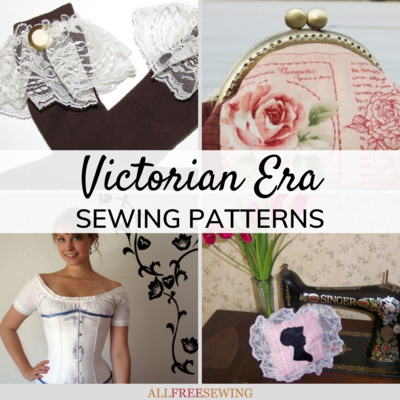In this image, we see a detailed collage focused on Victorian-era sewing, consisting of four quadrants with distinct elements. In the top left quadrant, there is a brown sleeve adorned with white, lacy, frilly trim and a golden loop. To the right, the top right quadrant displays a small, clasped purse featuring a golden frame and a rose fabric design intertwined with red diagrammatic sketches. In the lower left quadrant, a smiling Caucasian woman with blonde hair is dressed in a shiny, white silk corset over a white low-cut shirt, embodying Victorian elegance. The lower right quadrant showcases an antique Singer sewing machine, decorated with a floral gold trim, a pink pillow with white lacy edges, and a silhouette of a woman’s face on thin, light fabric. In the center of the collage, a semi-transparent white text box, with "Victorian Era" in cursive and "Sewing Patterns" in regular text, highlights the theme. At the bottom of the overall image, it reads "All Free Sewing."